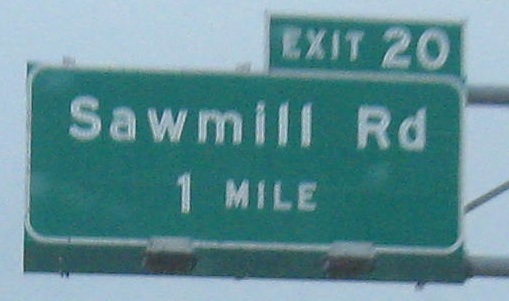A photograph captures a highway sign against an overcast blue sky. The sign, featuring a green background with a white border, reads "Sawmill Rd" with "Rd" abbreviated and is located one mile from the current position. In the upper right-hand corner, an attached green panel designates the exit number as "Exit 20" in white print. The sign is supported by cylindrical, silver-colored metal posts, positioned diagonally from the top right corner of the image, providing structural stability to the sign.